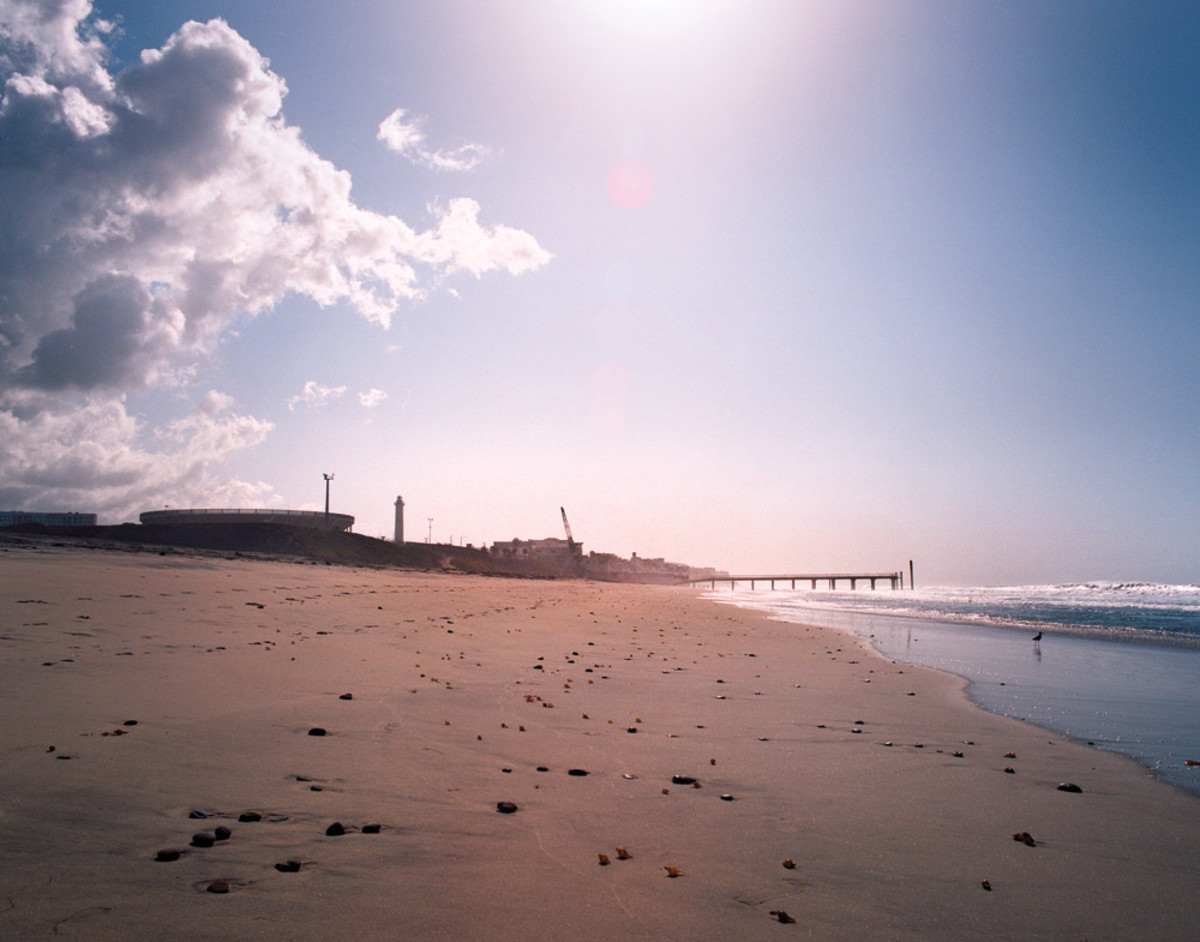This captivating color photograph captures a deserted beach during the daytime, featuring various striking elements. In the foreground, the medium gray sand stretches out, dotted with pebbles and litter, and merges into the wet shoreline on the right where a single small bird stands. To the right, gentle waves roll in, creating a clear delineation between the moist sand and the water. The background showcases a prominent pier jutting into the ocean, flanked on the left by a silhouette of short buildings and tall telephone poles. Above, the sky transitions from clear blue, especially in the upper right corner, to a pinkish hue near the horizon, crowned by a glaring sun partially visible near the center. On the left, a large mass of white, fluffy clouds contrasts with the mostly clear skies of the remaining two-thirds. This serene yet desolate scene is reminiscent of the Gulf Coast, possibly around Orange Beach, exuding a tranquil yet slightly mysterious ambiance.